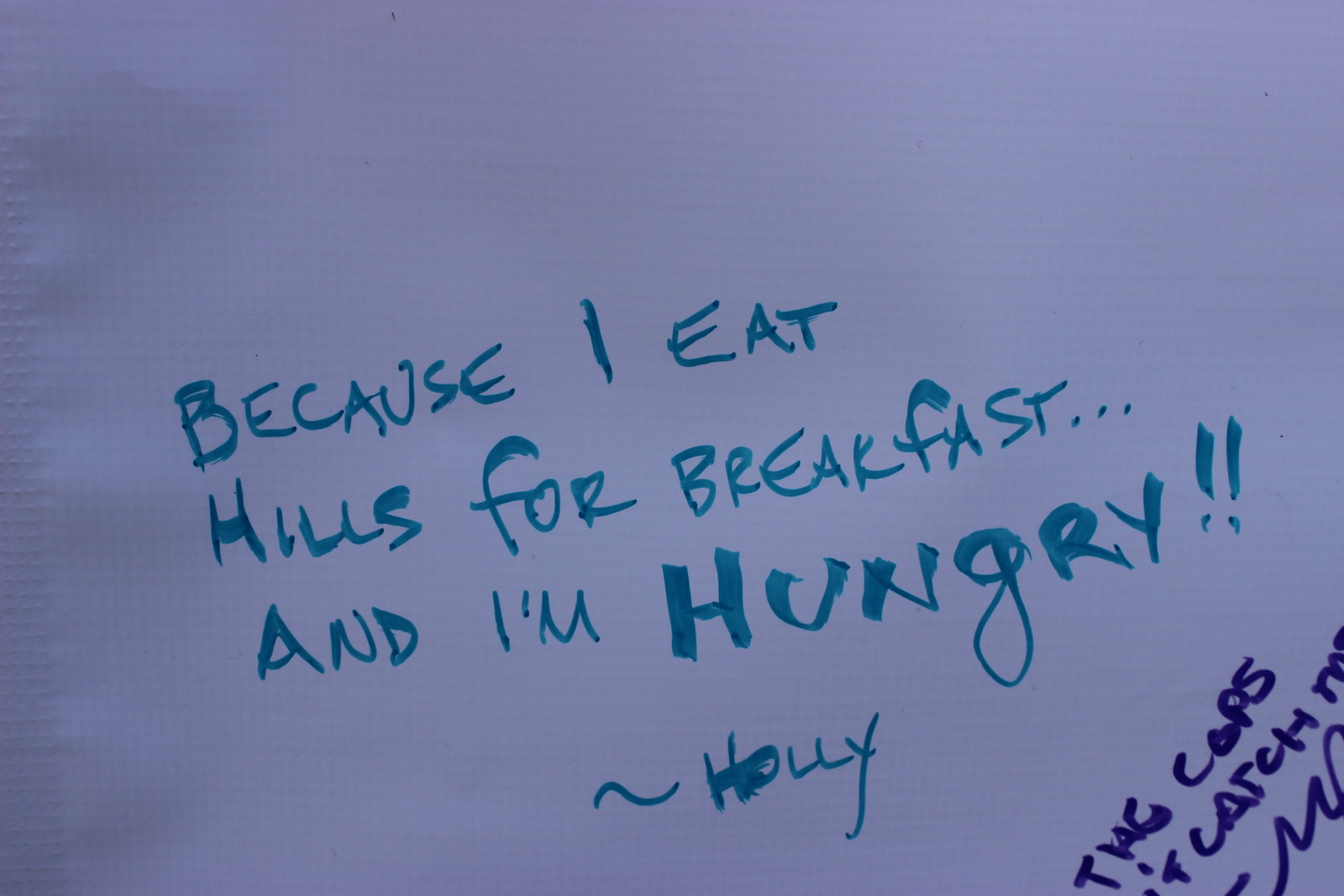The image is a photograph of a white sheet of paper with handwritten text in blue and purple markers. In the center of the page, written with a blue or turquoise felt pen, the text reads: "Because I eat hills for breakfast... and I'm hungry!!" This statement is signed by "Holly" in the same blue pen, positioned below the main text but slightly to the right. At the bottom right corner of the paper, written in a smaller purple font, is a partially visible quote or text that includes the words "THG Cops" and "catch," though the rest is cut off and unreadable. The overall layout features the main message prominently in the center, with additional elements in the lower right, creating a dynamic and somewhat mysterious composition.